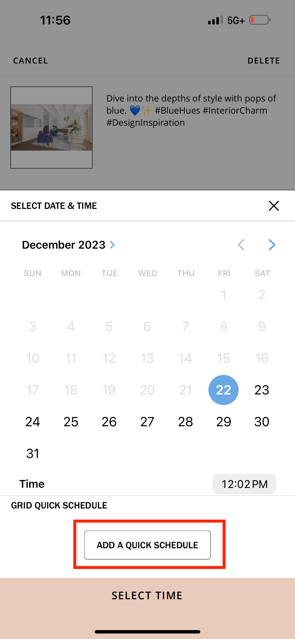The image is a detailed screenshot of a mobile phone interface, focusing on a scheduling tool. The foreground features a pop-up window for selecting a date and time in December 2023. The backdrop of the screen is grayed out to emphasize the pop-up.

The pop-up displays a calendar layout with the days of the week—Sunday, Monday, Tuesday, Wednesday, Thursday, Friday, and Saturday—arranged across the top. The dates for December are shown below, with the 22nd of December prominently highlighted in a blue circle, indicating the selected date.

Below the calendar, there's a section labeled "Time" with an input field where users can type in the desired time. The preset time in this field is 12:02 p.m.

Further down, the pop-up includes a section titled "Grid Quick Schedule" featuring an "Add Quick Schedule" button. This button is surrounded by a red annotation box, indicating that someone has marked it for emphasis.

At the very bottom of the pop-up, there’s another instruction, “Select Time.” The grayed-out background behind the pop-up shows an image accompanied by a caption that reads: "Dive into the depths of style with pops of blue 💙 ✨ #bluehues #interiorcharm #designinspiration".

The overall scene effectively captures a moment of scheduling an event while juxtaposing it with a stylish, inspirational background, highlighting both functionality and aesthetic appeal.